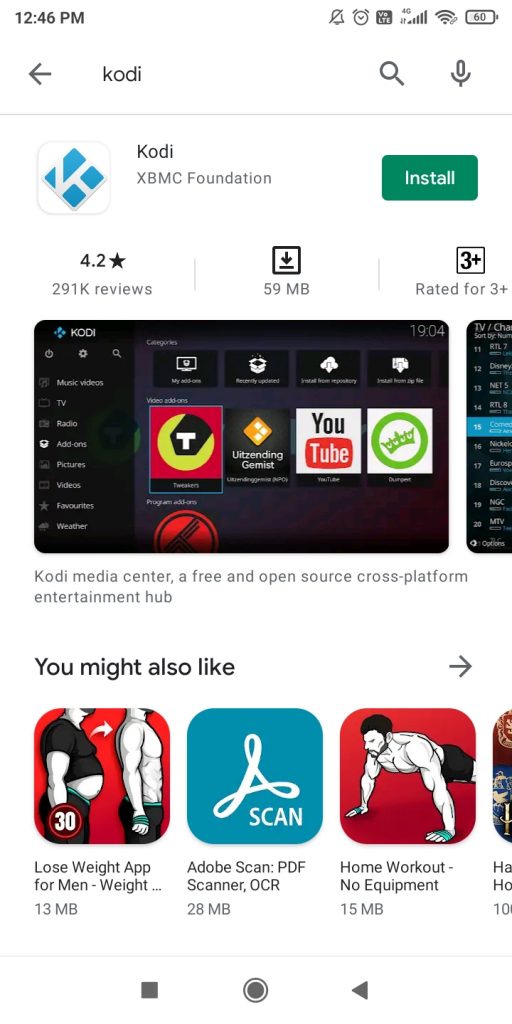The screenshot is a rectangular image captured from a smartphone, with the longer sides positioned vertically. The background is predominantly white. In the top left corner, there is a timestamp showing "12:46 PM" in gray text. The top right corner includes several icons: a bell, an alarm clock, a signal bar with full 4G reception depicted by five ascending bars, a signal strength indicator, and a battery icon displaying "60%."

Below this status bar, "Cody" is displayed in black text. A light gray line runs horizontally beneath the word "Cody." Further down, on the left side, there is an icon with a triangular silver "K" within a silver-bordered white square. To the right of this icon, the name "Cody" is written again, followed by "XBMC Foundation" underneath. On the far right side, there is a green rectangle with rounded corners containing the word "Install" in white text.

Continuing downwards, the image displays a rating of "4.2 stars" based on "291K reviews," and notes the app size as "59 MB."